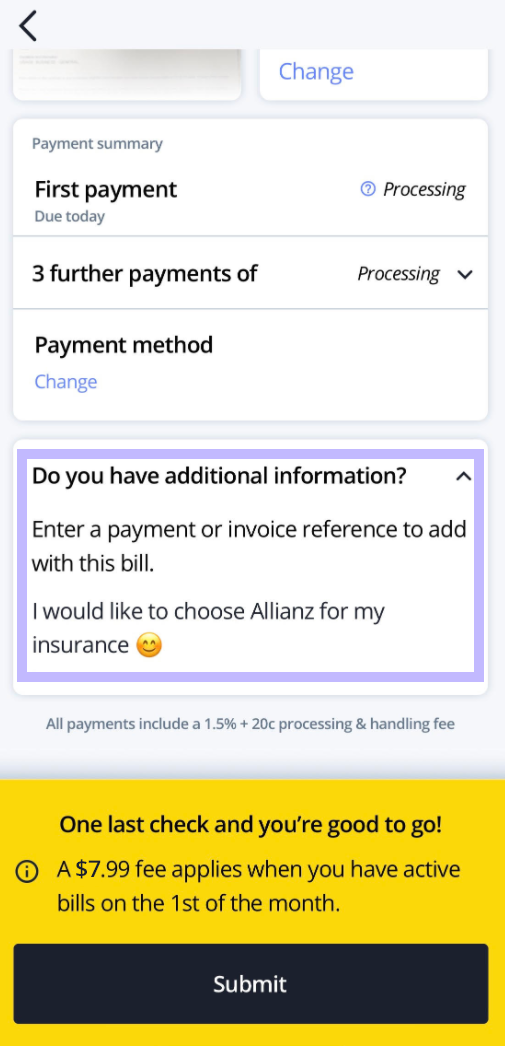The image depicts a vertically-oriented payment summary interface, likely designed for a mobile device. The layout features various sections, each clearly demarcated and color-coded for easier navigation.

- **Top Section:**
  - On the top left, a black arrow pointing to the left suggests a back navigation option.
  - Adjacent to this, there is a grayish area, followed by a white box with the word "Change" in blue.

- **Payment Summary:**
  - Below this is a white box titled "Payment Summary."
  - It lists details such as "First Payment," and "Due Today" in black text.
  - Towards the right side, it shows the status "Processing."
  - Further down, it mentions "Three further payments of" followed by "Processing."

- **Payment Method:**
  - Directly below the summary, another section details the "Payment Method."
  - The word "Change" appears in blue text, indicating an option to alter the payment method.

- **Additional Information:**
  - Another white box follows, headed by "Do you have additional information?" in black text.
  - An upward-facing arrow on the right side seems to be an interactive element.
  - It prompts the user to "Enter a payment or invoice reference to add with this bill."
  - An additional note states, "I would like to choose LENs for my insurance," accompanied by a smiley face emoji.

- **Border and Footer:**
  - Surrounding the interface is a purplish border, giving it a cohesive look.
  - At the bottom, a statement clarifies that "All payments include a 1.5% plus 20 cent processing and handling fee."
  - In a yellow box, a message reads, "One last check and you're good to go."
  - A note in this area specifies, "A $7.99 fee applies when you have active bills on the first of the month."
  - Finally, a prominent black button with the label "Submit" is present for finalizing the payment process.

This detailed caption aims to provide a comprehensive overview of the payment summary interface, highlighting its structure, content, and design elements for clarity.